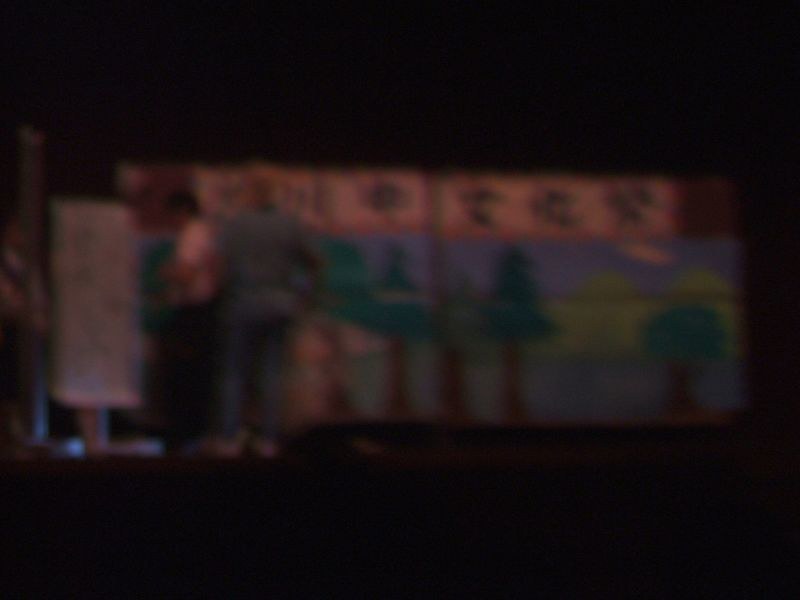In this blurred and dimly lit image, it is challenging to determine if the setting is indoors or outdoors at night. The top and bottom portions of the image are completely black, suggesting significant darkness. In the middle, a highly indistinct object appears, possibly a wall adorned with a painting or drawing. Though unclear, it seems to depict green trees with brown trunks set against a blue sky, dotted with white, cloud-like shapes.

On the left side of the image, two figures are discernible. One individual is dressed in a blue top paired with what could be blue jeans, appearing to face the painting directly. Next to them, another person is seen wearing a white top and dark bottoms. This second individual seems to be turned to the left, standing before a metal rectangular object, whose purpose or contents remain unclear. The overall scene is shrouded in low visibility, adding to the ambiguity of the surroundings.